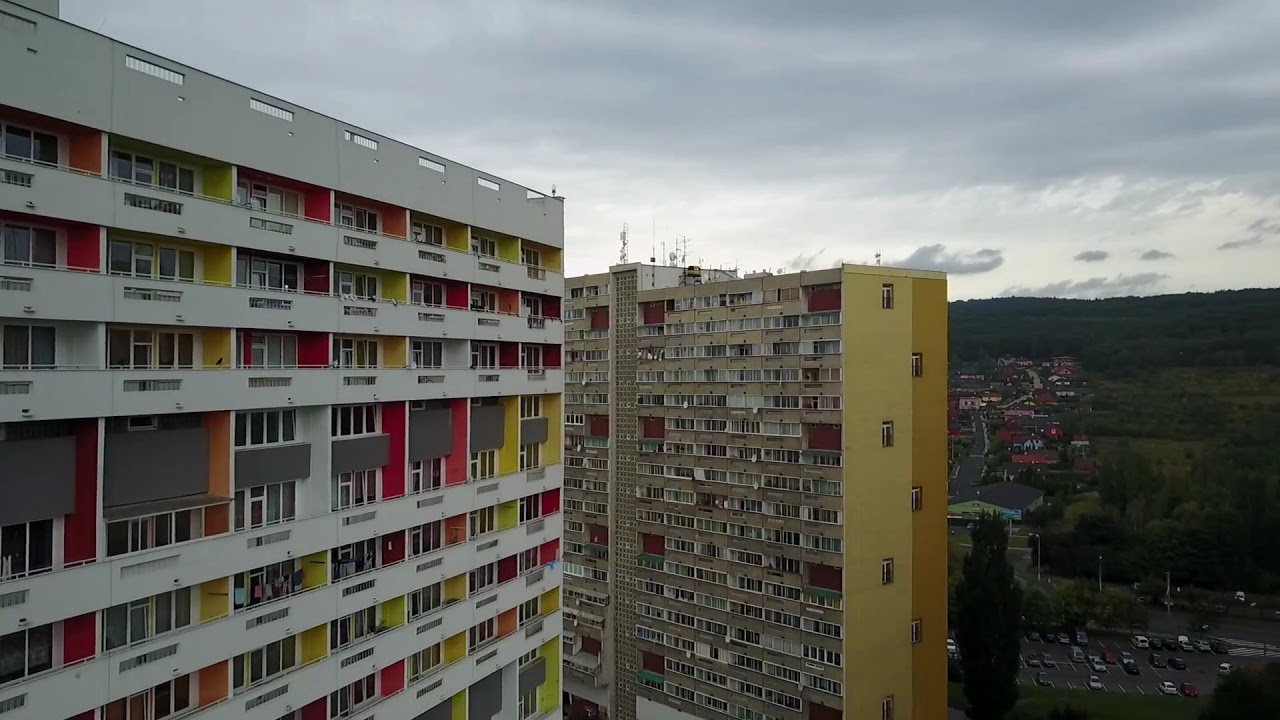This horizontally aligned, rectangular image, taken from approximately the 16th story of a building, captures a detailed urban landscape. On the left side, there is a very tall, multicolored apartment building with walls in shades of red, orange, pink, and yellow, segmented by horizontal white or light gray stone strips. Each unit features a balcony, with one showing a person towards the bottom left. The building appears to be around 20 stories high.

In the center, there is another towering condominium, predominantly brown with dark brown blended in and accented by yellow edges. It too boasts numerous balconies. Both buildings are strikingly high, seemingly over 20 stories, and the photo provides a close-up view of their upper sections.

The sky in the background is overcast, with a blanket of gray clouds and some brighter white ones. On the right side of the image, there is a landscape of green treetops and some smaller buildings, roads, and cars. At the bottom right corner, a small parking lot dotted with several tiny cars is visible.